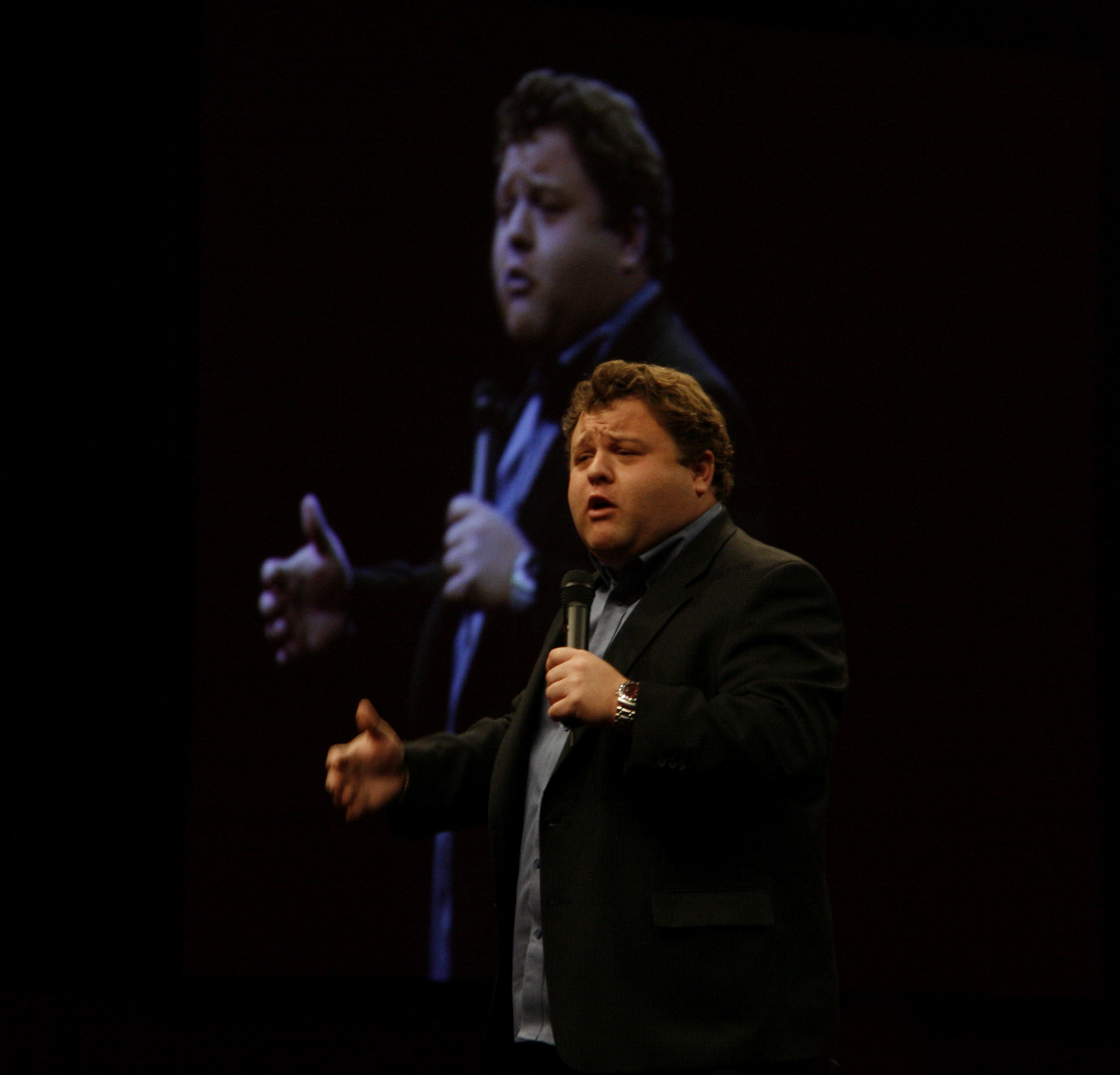The image captures a slightly heavyset man with chubby cheeks and medium-length, curly brown hair, wearing a black suit jacket left unbuttoned for a casual yet well-dressed look. Underneath, he dons a light blue, collared shirt that isn't tucked in, along with a silver watch adorning his left wrist. The man, who appears to be in his 20s or 30s, is holding a microphone in one hand while gesturing with the other, suggesting he might be speaking, singing, or performing to an unseen audience. The background is completely black, save for a large screen directly behind him that rebroadcasts his image in the same pose, creating a doubled visual of the man. His mouth is open mid-expression, heightening the sense of an active performance or presentation.